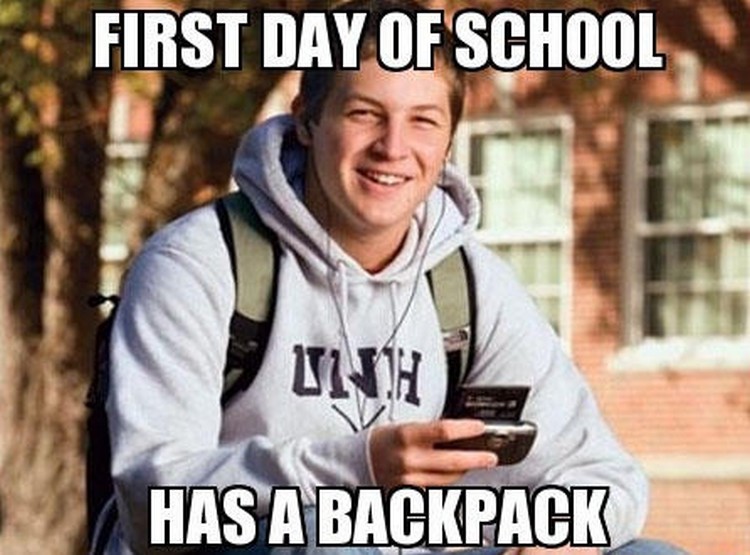The meme image features a smiling, white college student wearing a gray UNH hoodie, presumably from the University of New Hampshire. He has brown hair and wired earbuds placed in his ears. The student carries a light green North Face backpack, with visible grayish-green straps. In his hand, he holds an old-fashioned Sidekick phone with a distinctive flip-up screen and keyboard. The background, slightly blurred, features the image of a school building and a tree. The meme text is written in large, white, uppercase letters with a black border, stating "FIRST DAY OF SCHOOL" at the top and "HAS A BACKPACK" at the bottom, humorously implying the fleeting use of backpacks by college students after the initial excitement of the new school year.